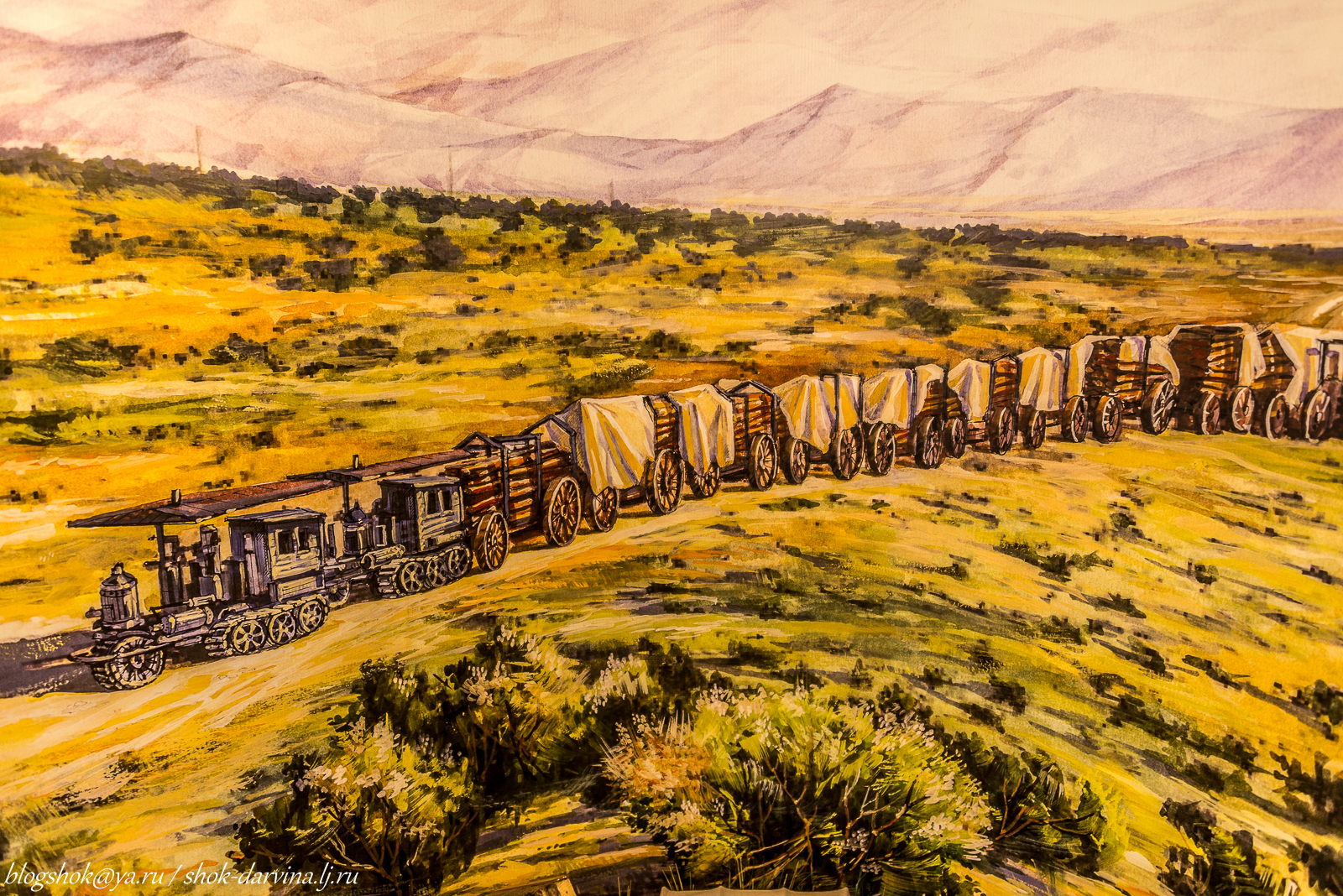This detailed painting depicts a historic Western scene featuring an old-school locomotive engine pulling a series of trolleys laden with lumber. The train, positioned prominently at the forefront, consists of two trams on tracks followed by multiple wooden carts covered with cloth. The ground is primarily a yellow-green hue, resembling a temperate desert climate, and is dotted with dark green bushes and sparse trees. The backdrop showcases sketches of mountainous designs with fading hilltops, indicating a daytime setting. At the bottom of the image, there is a watermark bearing the artist's username, adding a modern touch to this classic representation.